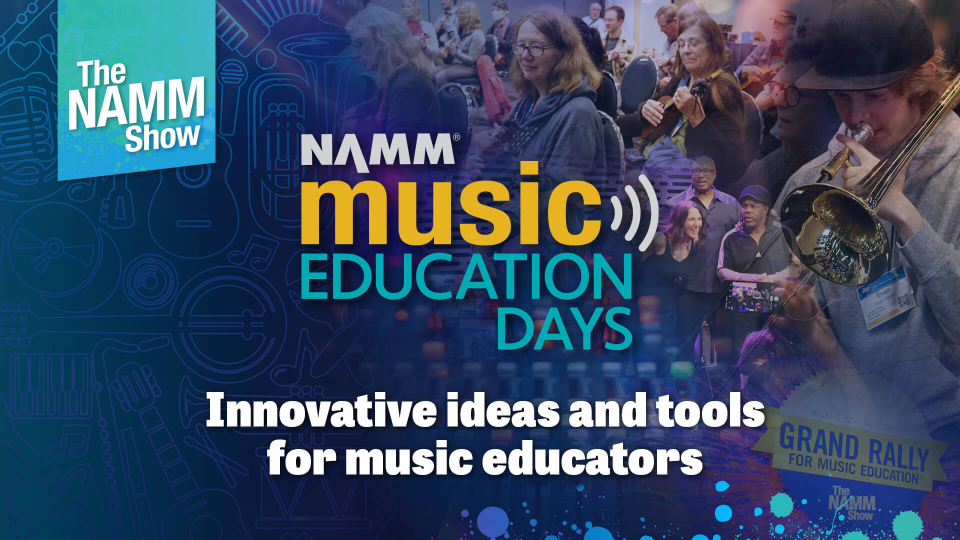The image appears to be an advertisement designed to promote an event. The layout is divided into two main sections: the left-hand side and the right-hand side.

The left-hand side of the image is dominated by a rich purple background. Centrally positioned within this purple backdrop is a small, light blue box with white text that reads "The NAMM Show." Directly below this, the word "NAMM" is prominently displayed in white letters. Below the word "NAMM," the word "Music" is featured in yellow, with design elements that mimic lines emanating outwards, resembling sound waves coming from a speaker. Further down, in green letters, are the words "Education Days," making the full text read as "NAMM Music Education Days." Beneath this headline, in white letters, is a subheading that says, "Innovative Ideas and Tools for Music Educators."

The right-hand side of the image is filled with a collage of photographs featuring a diverse array of people. These individuals represent various demographics and are engaged in musical activities, each holding different musical instruments. Among these, to the far right, there is a particularly large image of a person playing a bugle, distinguishable by the hat they are wearing. Other smaller insets show individuals with instruments like a mandolin, illustrating the communal and diverse nature of music-making.

In summary, the image is a vibrant and engaging promotional piece for "NAMM Music Education Days," highlighting its focus on innovative educational tools and ideas for music educators, and celebrating the diversity of people involved in music.